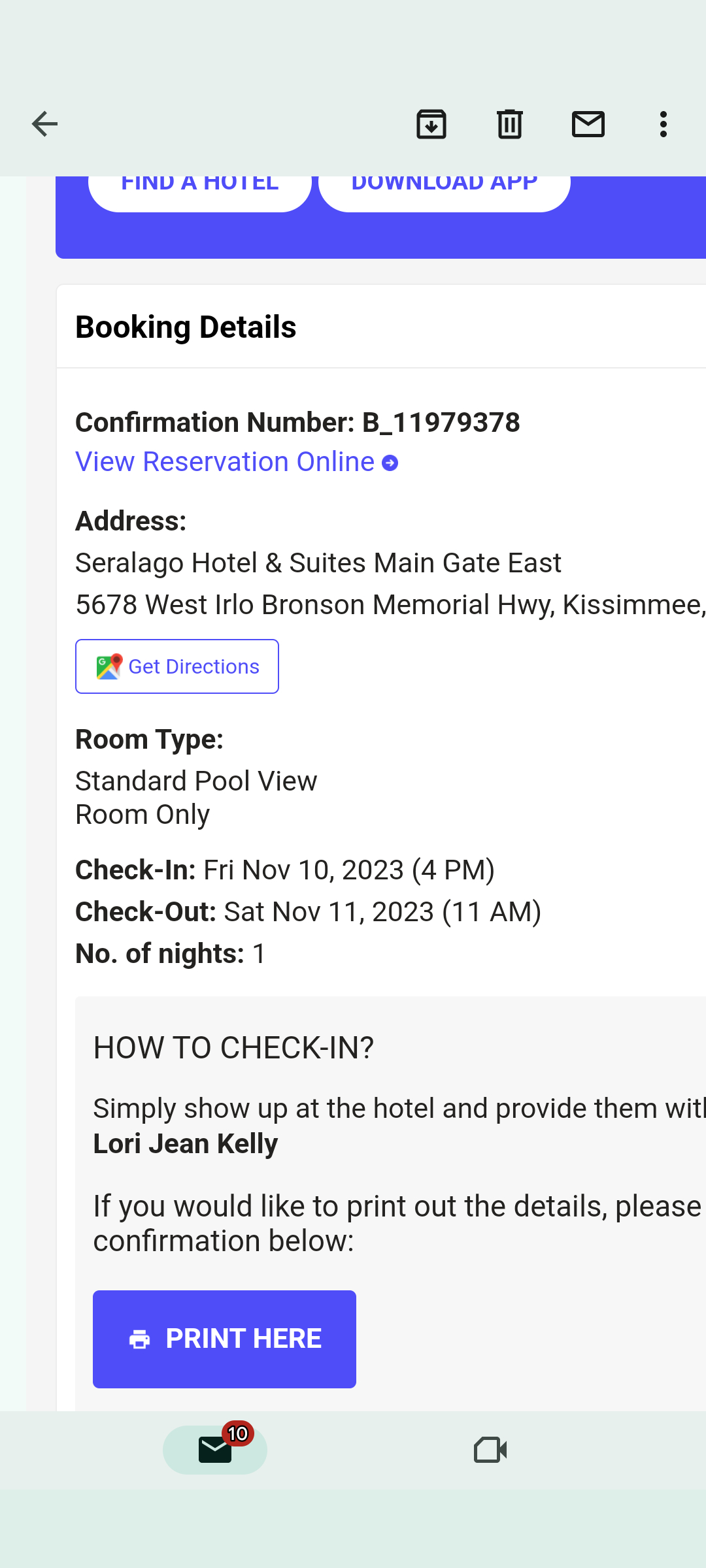A screenshot of a mobile phone screen displaying detailed booking information for a hotel reservation. The top section of the screen includes a mail icon, a three-dot menu icon, a trash can icon, and a download icon. 

The main content shows a partially obscured blue banner with buttons at the top, followed by a "Booking Details" header. Below this header, the confirmation number "B_11979378" is prominently displayed alongside a hyperlink that says "View reservation online."

Further down, the reservation details list the hotel's name and address: "Cerro Lago Hotel and Suites, Main Gate East, 5678 West Irlo Bronson Memorial Highway, Kissimmee." There is also an option to get directions via a clickable button.

Information on the room type specifies a "Standard Pool View Room Only," with check-in scheduled for Friday, November 10th, 2023, at 4:00 PM, and check-out on Saturday, November 11th, 2023, at 11:00 AM. The duration of the stay is listed as one night.

A gray box contains check-in instructions that are partly cut off, beginning with "Simply show up at the hotel and provide them with..." followed by the name "Laurie Jean Kelly." An additional note regarding printing details is also cut off, but a purple button labeled "Print Here" with an accompanying printer icon is visible.